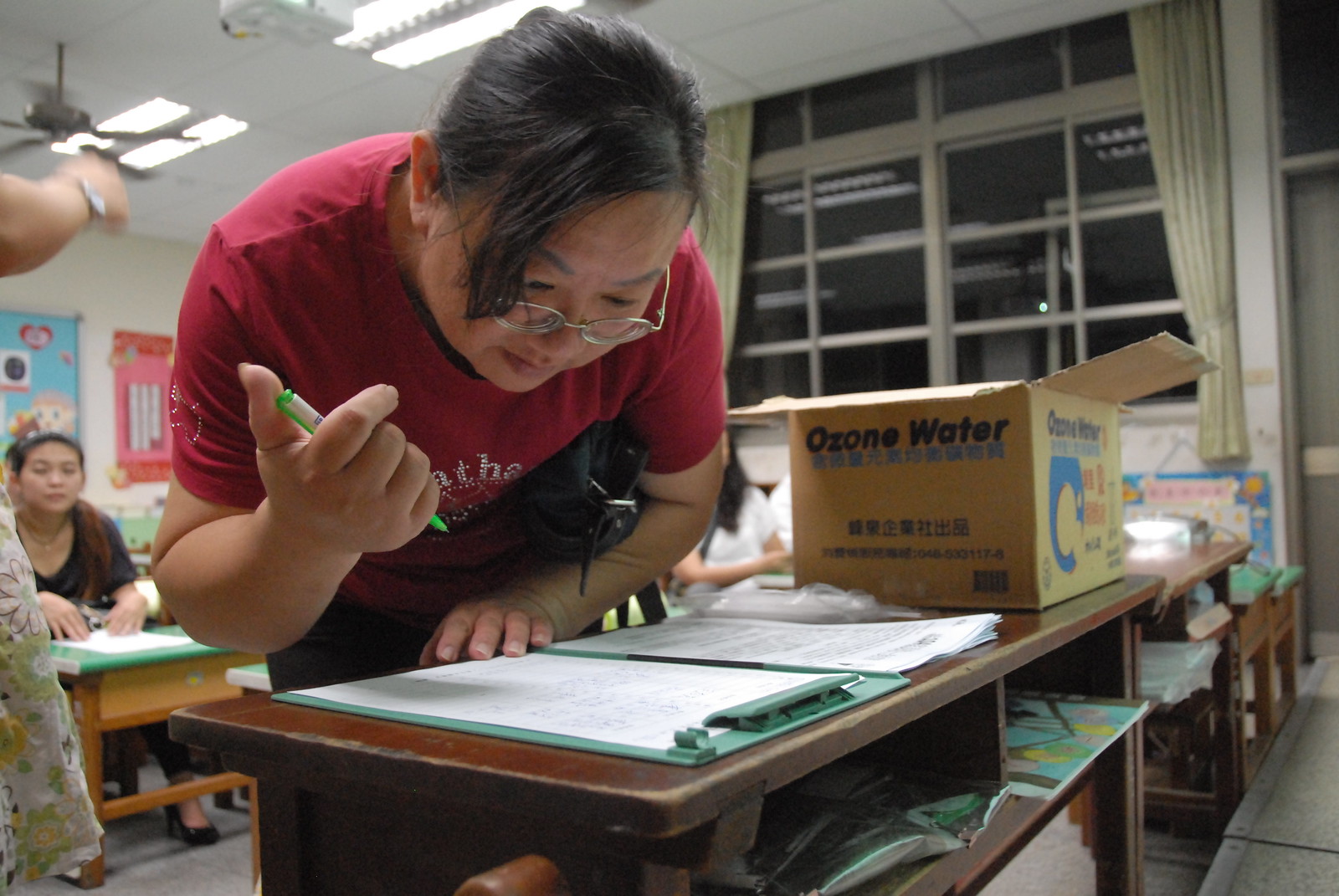In a classroom setting, an Asian woman is intently focused on signing a white piece of paper affixed to a light green clipboard. She is bent forward with her brown hair tied back, wearing circular glasses, and a red shirt. The clipboard rests on a dark brown desk that has the appearance of an open bookcase with visible storage underneath. The woman is clicking a green and white pen with her right hand, which hovers above the clipboard, while her left hand is steadied on the table. To her right, a cardboard box labeled "Ozone Water" with Chinese characters is prominently displayed. A navy blue-shirted woman sits in the background to the left, at a desk featuring a green surface and light brown wooden drawers. The scene is further detailed by the edge of a white skirt with floral patterns in green, yellow, and brown appearing at the bottom-left corner of the image. A sizable window with cream-colored shades and a ceiling fan projector can also be seen, indicating a well-lit classroom at nighttime.